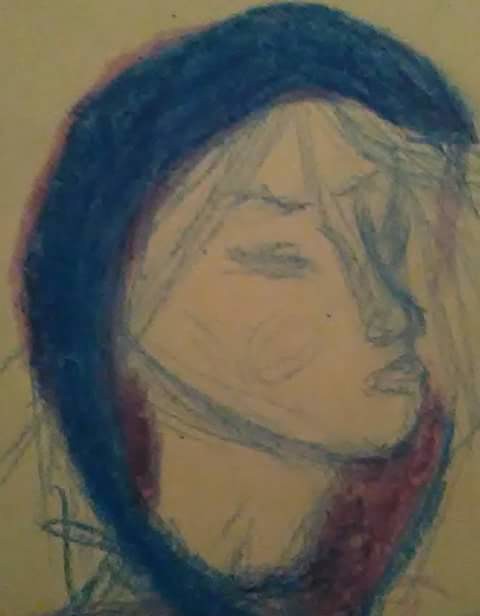This rectangular image, oriented with its longer dimension from top to bottom, showcases a photograph of a hand-drawn portrait. The drawing features a profile view of a person's face, meticulously rendered in what appears to be blue crayon or pencil. The subject's eye is closed, and detailed attention has been given to the contours of the nose, lips, jawline, and neck. A blue scarf, adorned with red highlights primarily on the bottom right, elegantly wraps around the head, starting at the top right, extending to the middle top, and descending to the left side before nestling under the chin. The drawn figure also displays hair flowing from the head, completing the serene and composed appearance of the portrait.